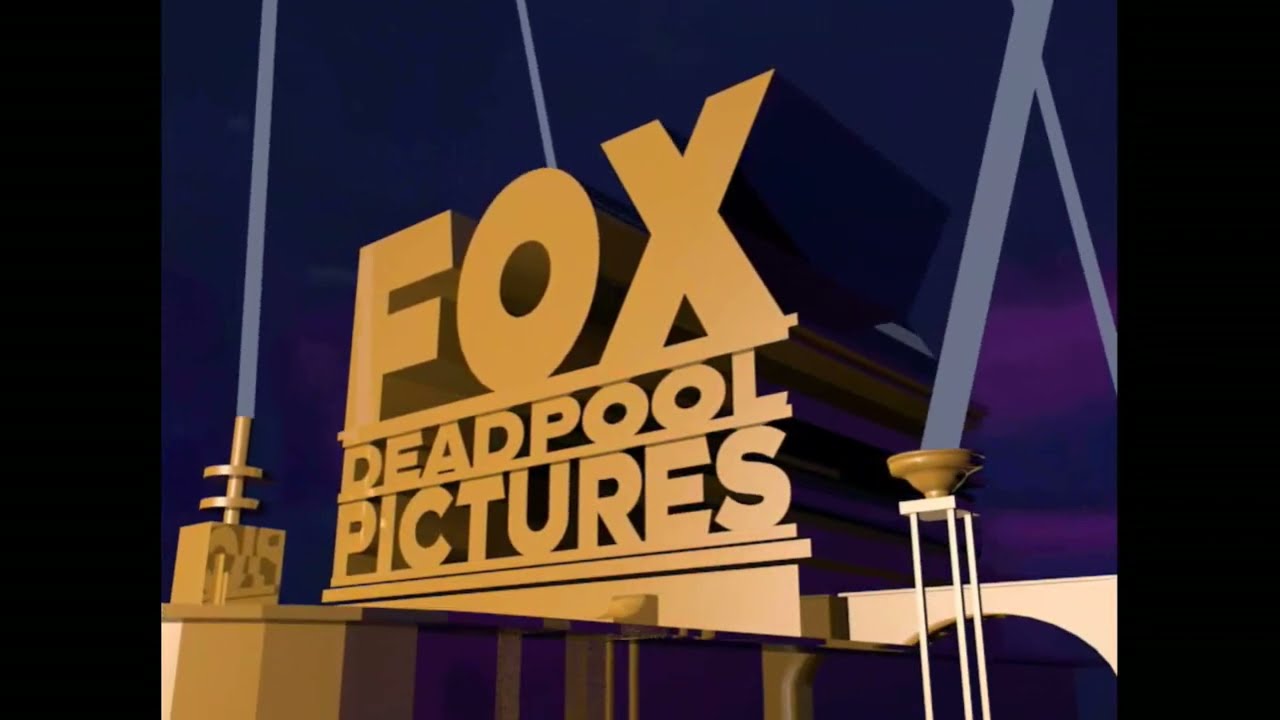The image appears to be a screen grab from a movie or television screen with black borders on both the right and left. It prominently features a cartoon-style logo set against a purple night sky with streaks of light gray, symbolizing searchlights, piercing through the sky. At the center of the image, there is a gold platform supporting three-dimensional, gold block lettering that reads "FOX" in large, bold capital letters, and beneath it, in smaller font, "DEADPOOL PICTURES." These words are angled from left to right towards the viewer. The distinctive elements of the scene, reminiscent of a classic movie studio logo, are the numerous searchlights positioned at ground level. These fixtures are aimed skyward, reminiscent of the dramatic illumination seen at a movie premiere. On the bottom right of the image, there is a golden cube supporting one of the searchlights, adding to the grandeur of the visual theme. The overall color palette combines deep purple and blue hues for the sky, enhancing the contrast with the brilliant gold lettering and light fixtures.